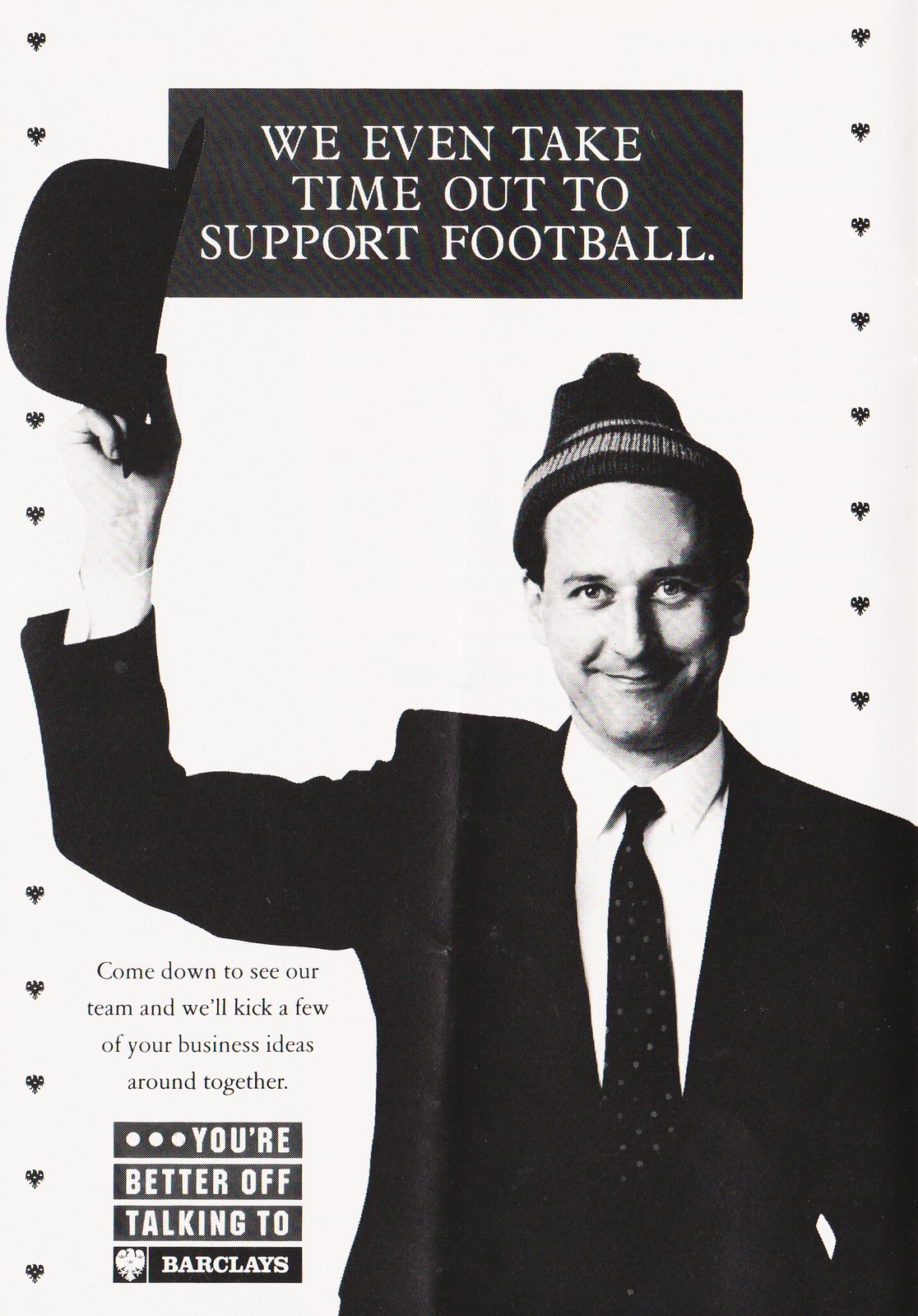This vintage black-and-white print publication, likely a flyer or poster, features a smiling man standing at the bottom right corner, dressed in a black suit, white shirt, and black tie. He is holding a black top hat in his right hand, raised above his shoulder, while wearing a knitted black beanie on his head. The image is set against a light gray background and is punctuated with graphic design and typography reminiscent of vintage style.

At the top of the poster, within a black rectangle, white text in uppercase reads: "We even take time out to support football." At the bottom left, below the man’s arm, more text reads: "Come down to see our team and we'll kick a few of your business ideas around together." Underneath this, bold white lettering on three black stripes declares: "You're better off talking to Barclays." To the left of the word "Barclays," there is a round logo symbol, and similar logos run along the left and right margins of the image. This detailed composition combines photography with graphic design, making it a striking visual piece.